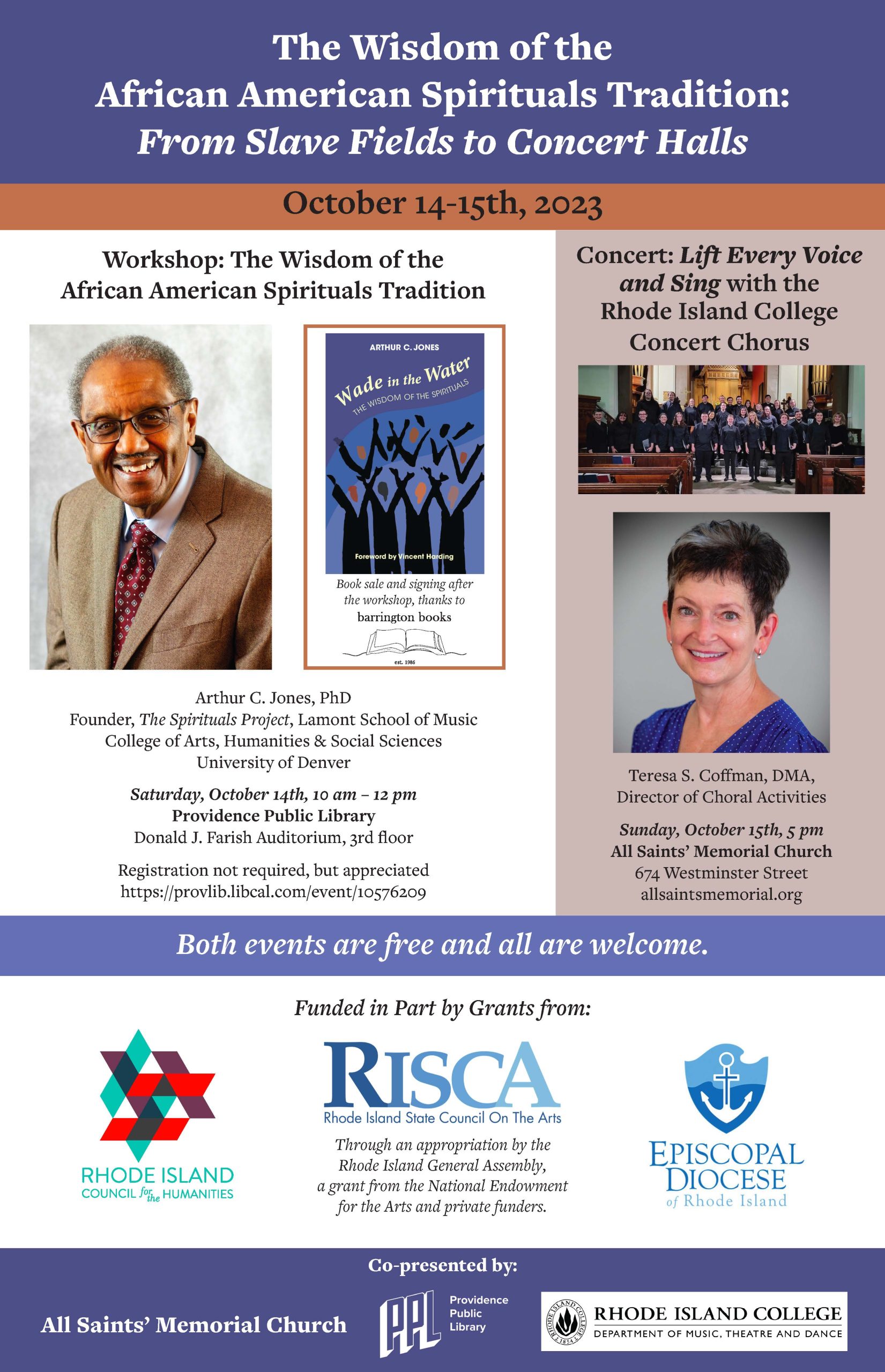This is a digitally created flyer for an event focusing on the wisdom of the African American spirituals tradition, spanning from slave fields to concert halls. The event takes place on October 14-15, 2023. The top section of the poster features the title in white text on a blue background, followed by the event dates and details about the workshop and concert, encapsulated in an orange border. The workshop is titled "The Wisdom of the African American Spirituals Tradition" and will be led by Arthur C. Jones, Ph.D., founder of the Spirituals Project, on October 14th, from 10 a.m. to 12 p.m. at Providence Public Library's Donald J. Farish Auditorium on the third floor. 

An image of Dr. Jones, an African American man in a brown suit and red tie, smiling and wearing glasses, is featured alongside a brochure titled "Wade in the Water: The Wisdom of the Spirituals." The concert, "Lift Every Voice and Sing," will take place on October 15th at 5 p.m. at All Saints Memorial Church on 674 Westminster Street, directed by Teresa S. Kauffman, who is depicted with short hair, fair skin, and a blue v-neck shirt.

The flyer includes a section indicating that both events are free and open to the public, showcased in white text on a blue border. The sponsors at the bottom include the Rhode Island College Concert Chorus, All Saints Memorial Church, Rhode Island College (RIC), RISCA, Rhode Island Council for the Humanities, and the Episcopal Diocese of Rhode Island.